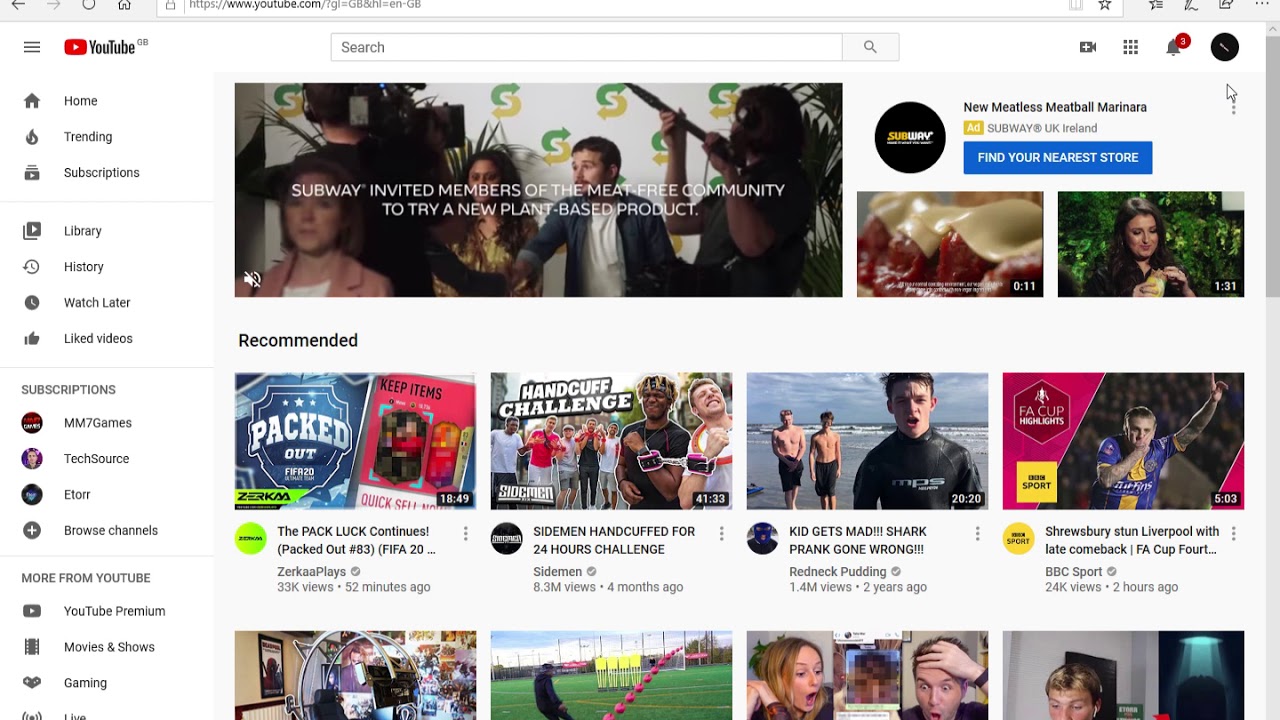This is a detailed description of the homepage for YouTube's Great Britain website. At the very top left corner beneath the address bar and browser buttons, the YouTube logo is labeled specifically as "YouTube GB," indicating that this is the Great Britain version of the site. Centrally located at the top is a search bar, while on the right side, there are several buttons. Notably, there's a bell icon with a notification indicator—a red circle with the white number "3" inside it. On the far right, the user's avatar is displayed, featuring a black background with a white line through it. 

An advertisement for Subway is prominently displayed, promoting their new meatless meatball marinara. It includes the text "Subway UK Ireland" and a blue button with white text that reads "Find your nearest store." Below the text, there are video clips with timestamps, likely showcasing the product, and the main image appears to be of a man being interviewed, perhaps after winning an award or attending an event. The caption below this visual states, "Subway invited members of the meat-free community to try a new plant-based product."

To the left, the typical YouTube menu bar is present, while on the right is the main content area with thumbnails for various recommended videos. Two rows of video thumbnails can be seen, although the bottom row is partially cut off. Each row contains four video thumbnails arranged in four columns.